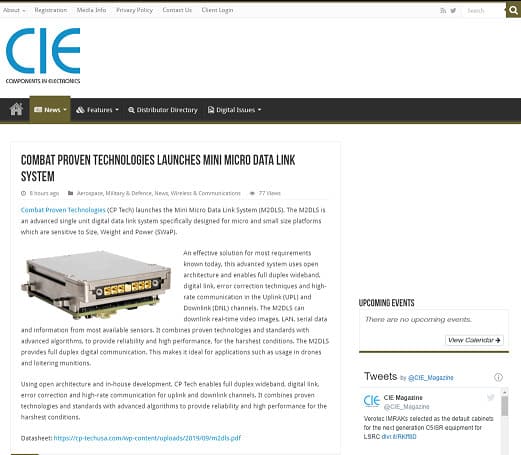The image is a square screenshot of a webpage displayed against a white background. In the upper left corner, there are several navigation options listed side by side, including "About," "Registration," "More," and "Mobile Info," though they are faint and hard to read. Next to these, there is a "Contact Us" link followed by a "Client Logo," "Log In," and "Client Log In" labels. On the far right of this navigation bar is a small search field. 

Directly beneath this line of navigation tabs, in large, prominent letters, is the "CIE" logo, representing Components in Electronics. Below the logo, a narrow black horizontal banner spans across the screen featuring several categories: "Home" (marked with an icon), "News" (highlighted as the current selection), "Features," "Distributor Directory," and "Digital Issues."

Further down, a news article is displayed with the headline "Combat Proven Technologies Launches Mini-Micro Data Link System." Though the article's text is too small to discern, there is an accompanying image that shows the component related to the news headline.